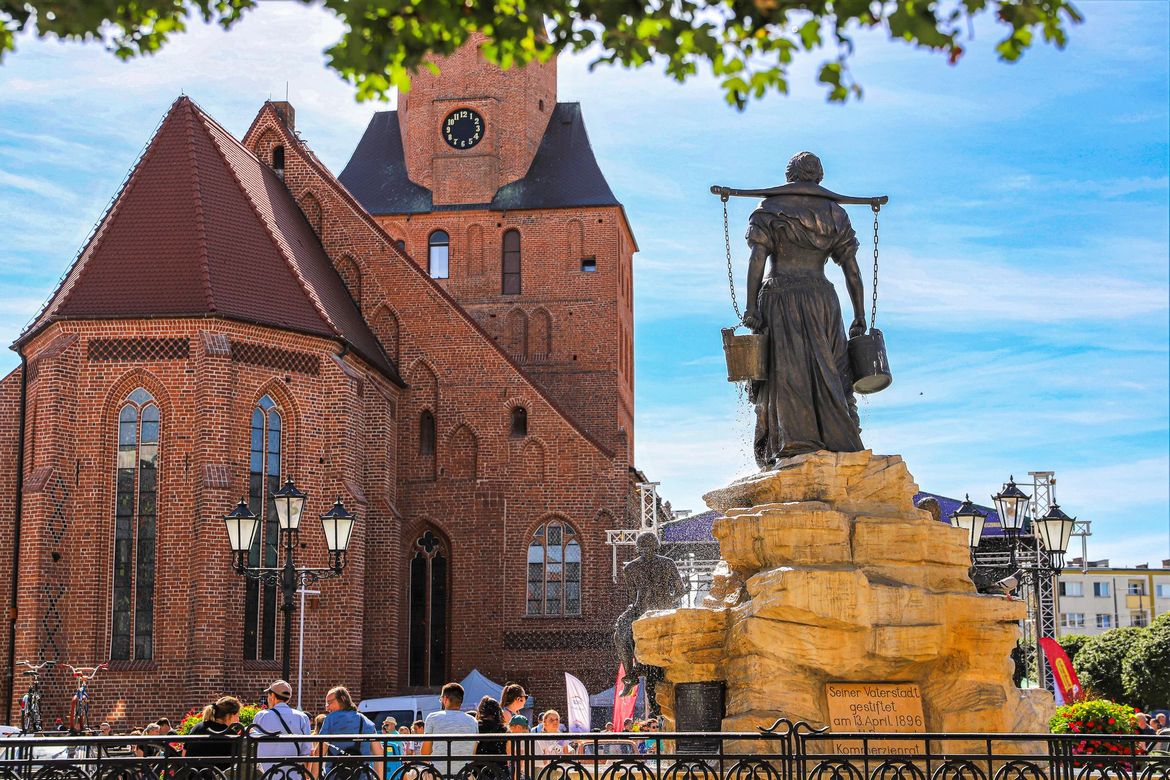This color photograph captures an outdoor scene with intricate details. Dominating the right-center is a naturalistic, orange-colored stone pedestal, topped with a bronze statue of a woman facing away from us towards the left. She is depicted carrying two buckets, each hanging from a chain attached to a yoke across her neck, with water visibly spilling from them, indicating it functions as a live fountain. To the left of this statue, slightly down below, another statue sits with its feet dangling off the rocky outcrop.

In the background to the left, there is a significant red brick building resembling a church, featuring tall, skinny, gothic-shaped stained glass windows and a steeple with an apse in the front. At the far end of the building, a black and gold clock tower rises prominently. The structure's dark red shingled roof contrasts with the blue sky dotted with white clouds above.

In the immediate foreground is a low black wrought iron fence, which frames part of the scene. Between the statue and the church, there's a street with a sidewalk, along which a crowd of people stands, likely attending an event near the church. The photo hints at the vibrant life of the place, with the statue’s plaque dated April 13, 1896, and inscribed in Polish, adding a historical touch to this picturesque setting.